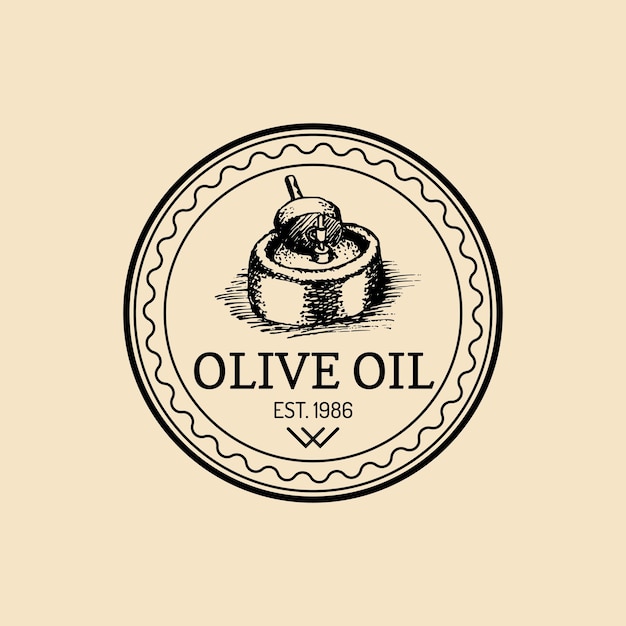The image depicts a detailed, vintage-style logo for an olive oil company, established in 1986. The logo is rendered entirely in black on a warm tan, almost beige, background. At the center of the design is a medallion-like emblem composed of concentric circles with varying line widths and styles, including wavy and straight lines that create a textured border. Inside the circular frame is an illustration resembling a manual nut grinder, contributing to an old-fashioned, pen-and-ink aesthetic. Below this central image, the words "OLIVE OIL" are prominently displayed in all capital letters, with "established 1986" inscribed underneath, flanked by overlapping V's that form a stylized W.